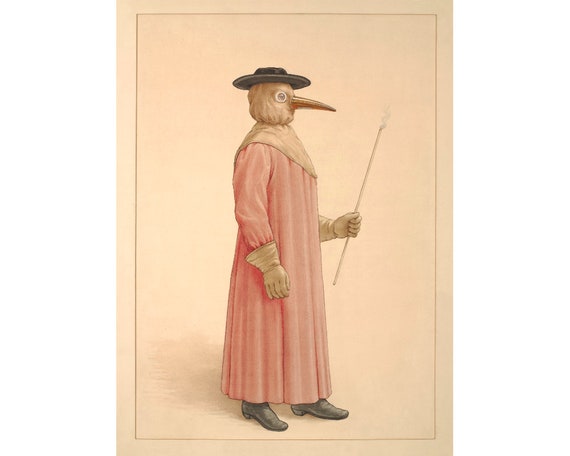This detailed illustration depicts a figure reminiscent of a character from the era of the Black Plague, possibly a plague doctor, or a fantasy scarecrow. The figure is shown in profile, adorned in a long pink robe and beige gloves that extend to the forearms. It wears a distinctive black hat over a brown head mask that covers the head, shoulders, and chest, featuring a prominently tapered, elongated beak. The eyes are large and round, adding to the character's striking appearance. Black shoes complete the ensemble. In its left hand, it holds a thin stick or possibly a lit torch or incense stick, with the suggestion of smoke adding to the eerie semblance. The scene is drawn on light brown paper or canvas, bordered with darker brown lines. The background is a soft pink, enhancing the figure's presence. The drawing style appears to use colored pencil or watercolor, contributing to the textured and aged look of the piece.